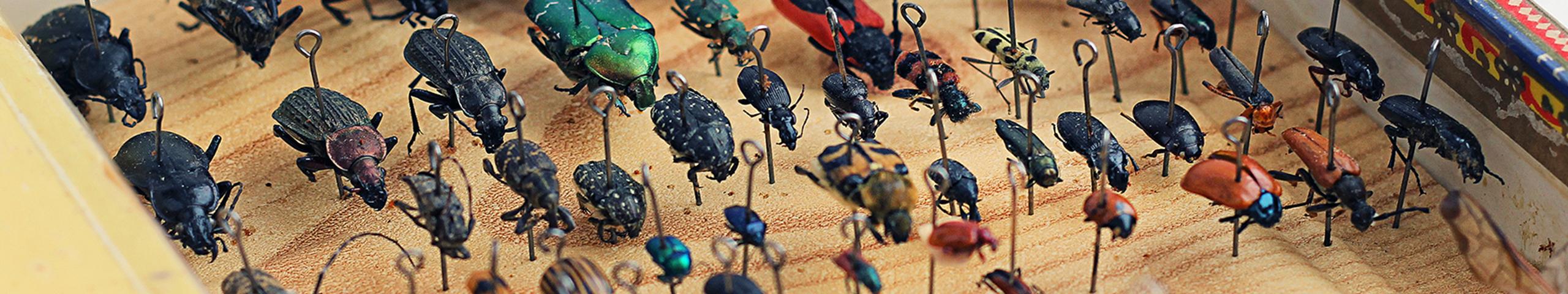The image depicts a panoramic view of a meticulously arranged collection of insects pinned onto a textured, brown cork board with a green hue. The collection primarily consists of various beetles, showcasing a range of sizes and colors. Most insects have black bodies, with some displaying shiny green exteriors and others in orange or reddish hues. In addition to beetles, the collection includes a few small flies and roaches. The photograph captures the systematic arrangement of these insect specimens, suggesting a detailed study or examination. The aspect ratio of the image appears to be narrow and wide, emphasizing the extensive and organized nature of the bug collection.